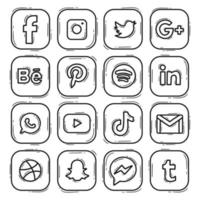This image features a hand-drawn, black-and-white 4x4 grid of well-known social media and app icons. Each icon is rendered in a minimalistic, stylized manner.

In the first row, from left to right, the icons are: Facebook (an ‘F’), Instagram (a camera outline), Twitter (a bird), and Google Plus (a ‘G+’). The second row includes: Behance (a capital ‘B’ with a lowercase ‘e’ and a line above it), Pinterest (a cursive ‘P’), Spotify (a circle with sound waves), and LinkedIn (a lowercase 'in'). The third row features: WhatsApp (a speech bubble with a telephone receiver), YouTube (a rectangle with a right-facing triangle), TikTok (a musical note shaped like a ‘J’ with a tilted top), and Gmail (an envelope). The final row displays: Dribbble (a basketball icon), Snapchat (a ghost with arms down), Facebook Messenger (a speech bubble with a lightning bolt), and Tumblr (a lowercase ‘t’).

These icons, representing familiar apps, seem hand-drawn and convey a simplistic style, devoid of color, suggesting perhaps a doodle or sketch meant to mimic typical smartphone app layouts.